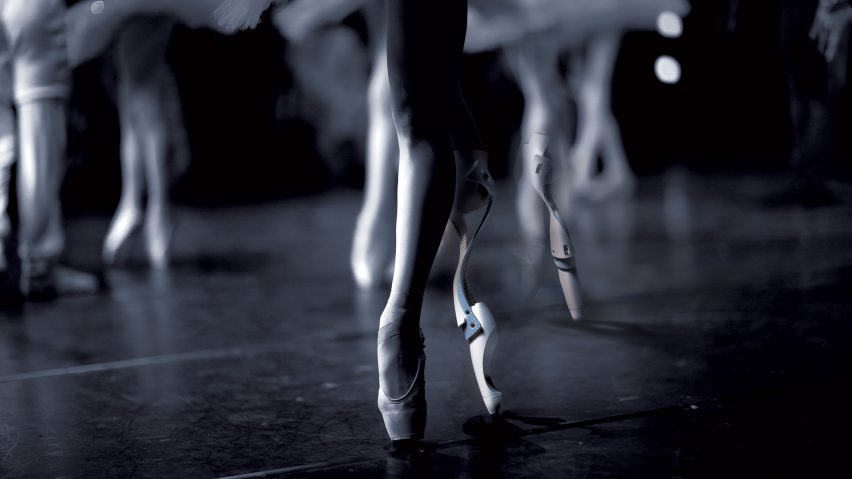The black and white photograph captures a striking and futuristic scene centered around a group of ballet dancers. The primary focus is a woman's slender, muscular leg, adorned with a ballerina's toe shoe, balanced delicately on tiptoe. Her other leg is a metallic prosthetic, demonstrating her elegance and resilience. Surrounding her are other dancers' legs, primarily shown from just above the knee down, with each dancer in various ballet poses on a glossy black stage floor. The image is slightly blurred, emphasizing the central figure's leg but still revealing other dancers, some standing on pointe, and others with feet flat. The dancers wear pale-colored ballet shoes and white dance costumes, adding to the monochromatic and polished aesthetic of the scene.